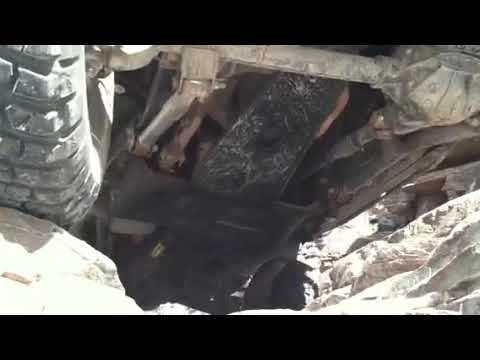The image is framed by black rectangular borders at the top and bottom, collectively occupying about one-fifth of the picture. It depicts the undercarriage of a vehicle, likely a truck or possibly a dune buggy. On the left side, a large wheel is visible, suggesting the vehicle is off-road. Surrounding the vehicle are jagged, tan-colored rocks, contributing to a rugged, rocky canyon setting. The bottom part of the truck is detailed with various mechanical components, including an axle and supports, metal protrusions, pipes, gears, and a significant skid plate protecting the engine. This underside view emphasizes heavy, black metallic structures, enhancing the impression of a robust, all-terrain vehicle. The angle suggests the camera is positioned below, capturing the vehicle from underneath as it traverses the rough landscape.